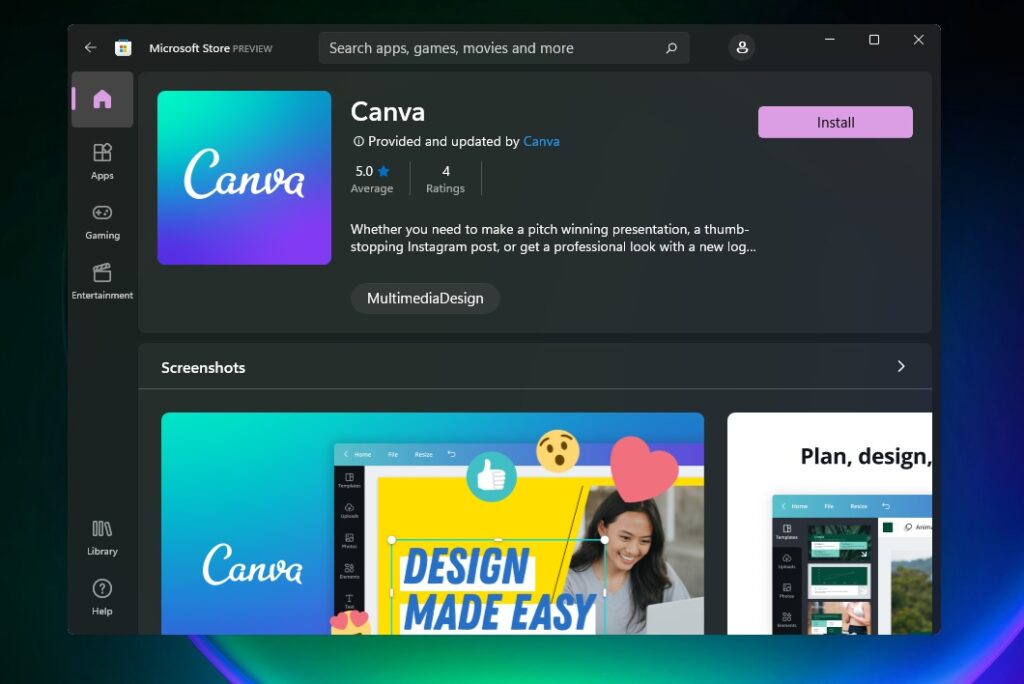**Detailed Caption:**

The screenshot showcases the Microsoft Store interface in dark mode, with black dialog boxes and dark gray accents, which indicates a nighttime or low-light browsing preference. The user is not logged into a specific profile, as evidenced by the absence of a user icon or name. Prominently displayed in the store's search bar are options to look for apps, games, movies, and more.

The highlighted application in the screenshot is Canva. It features a perfect five-star rating based on four reviews. The initial part of Canva’s description is visible, enticing users with promises of tools for creating pitch-winning presentations, eye-catching Instagram posts, and professional designs, with the full text truncating for a more detailed description not shown in the screenshot. An 'Install' button is available for initiating the download.

Below the description, there are preview images of Canva that exhibit its versatile uses, ranging from photo editing to various other creative functionalities. The overall layout implies that the user is considering installing Canva, evidenced by the position and emphasis on the application in the interface.